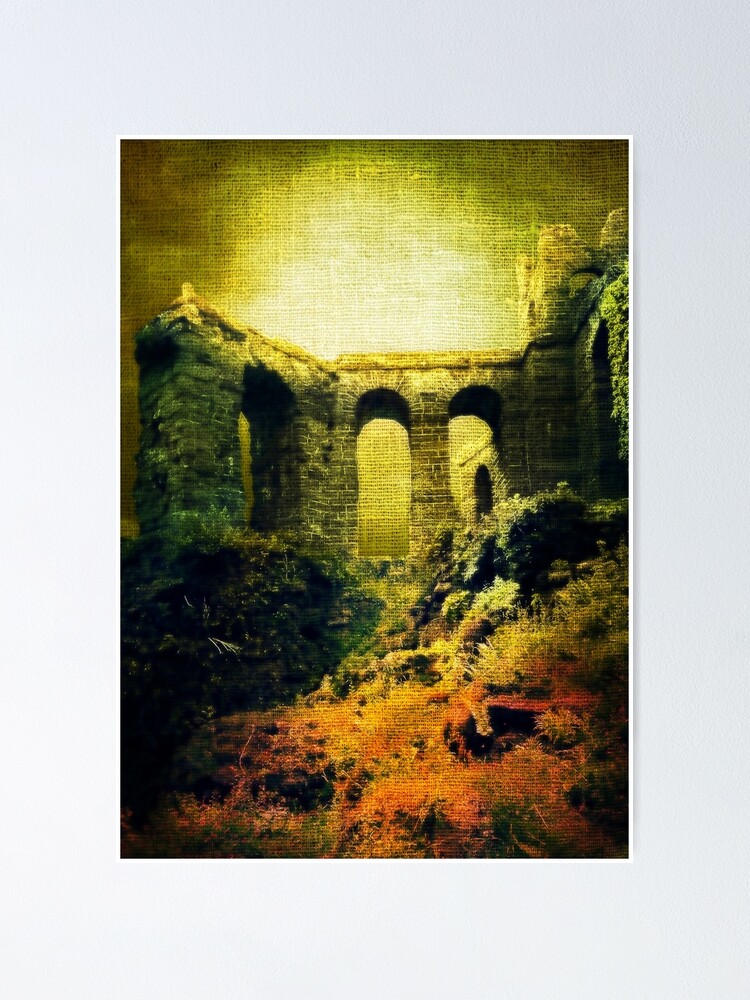The image is a framed print that convincingly replicates the look of an oil painting, depicting an ancient stone building with a classical aesthetic. Dominating the structure are three tall, imposing arches that extend from a cliffside, suggestive of a damaged aqueduct. The partially collapsed state of the aqueduct indicates its historical ruin. Surrounding the building, vibrant foliage of various hues—green, orange, yellow, and brown—intermingles with scattered rocks and brambles. The sky above is a striking mixture of bright yellow and white, resembling the sun at either a sunrise or sunset, surrounded by shadows and fading into darkness at the corners. This complex interplay of natural and architectural elements conveys a historical and picturesque setting, elevated by the detailed and color-rich portrayal. The entire scene is set against a gray background, enhancing the focus on the vivid and intricate artwork.